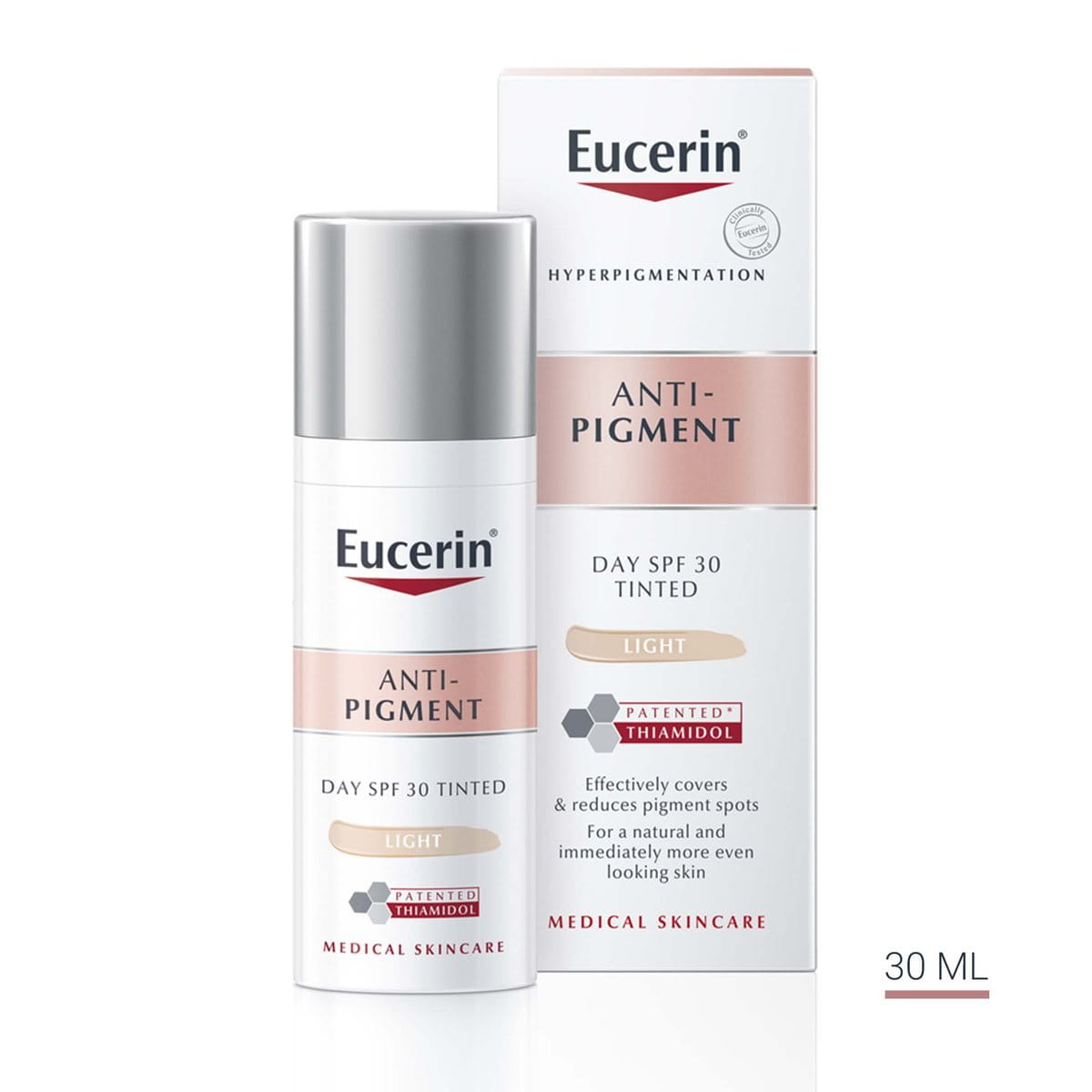This photo features a detailed view of a bottle of Eucerin Anti-Pigment Day SPF 30 Tinted skincare product and its accompanying box. The white bottle with a gray cap prominently displays the Eucerin logo, a small red upturned triangle beneath it, and the word "Anti-Pigment" in bold on a pink band around the middle. Below this, the text "Day SPF 30 Tinted" is written in black, followed by an image of a light-colored cream streak and the word "Light" in white. The next section features three interconnected hexagons alongside the phrase "Patented Thiamidol," where "Patented" is in red text and "Thiamidol" is in white text on a red background. At the bottom, it states "Medical Skin Care" in red. The box mirrors the bottle's design elements but includes additional text below the "Patented Thiamidol" logo: "Effectively covers and reduces pigment spots for a natural and immediately more even-looking skin." On the box, there's also a logo near the Eucerin branding with the term "Hyperpigmentation" underneath it, resembling an approval stamp. In the lower right of both the box and bottle, the quantity is specified as 30 milliliters with a red underline.